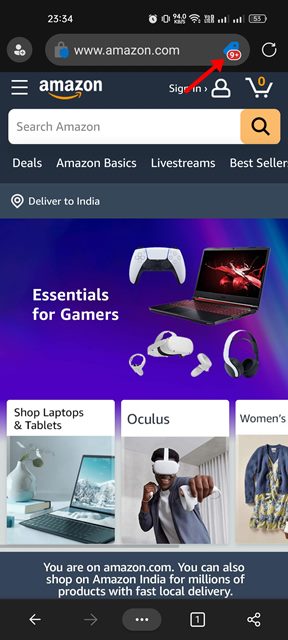This image is a screenshot taken from a phone displaying the Amazon website's homepage. At the top of the screenshot, the military time is shown as 23:34 hours. On the right-hand side of the status bar, several icons are visible: a clock, Wi-Fi signal indicator, battery level at 55%, and another icon that is not clearly identified.

Directly beneath the status bar, there is a search bar featuring Amazon's URL (www.amazon.com), alongside a red arrow pointing to a "9+" which likely indicates notifications or deals. The search bar also includes the Amazon logo with its signature smile and, beneath it, another search bar containing a magnifying glass icon within an orange box.

The main section of the homepage highlights "Essentials for Gamers," showcasing various gaming items such as a laptop, a controller, and what appears to be a Meta or Oculus VR headset. Below these items, there are tabs for different categories, including "Shop Laptops and Tablets," featuring images of a laptop and an Oculus headset. The first tab in the row, partially cut off, appears to be for women's merchandise.

At the bottom of the screenshot, there is a note indicating that the user is browsing Amazon.com, with some follow-up information partially visible but cut off.